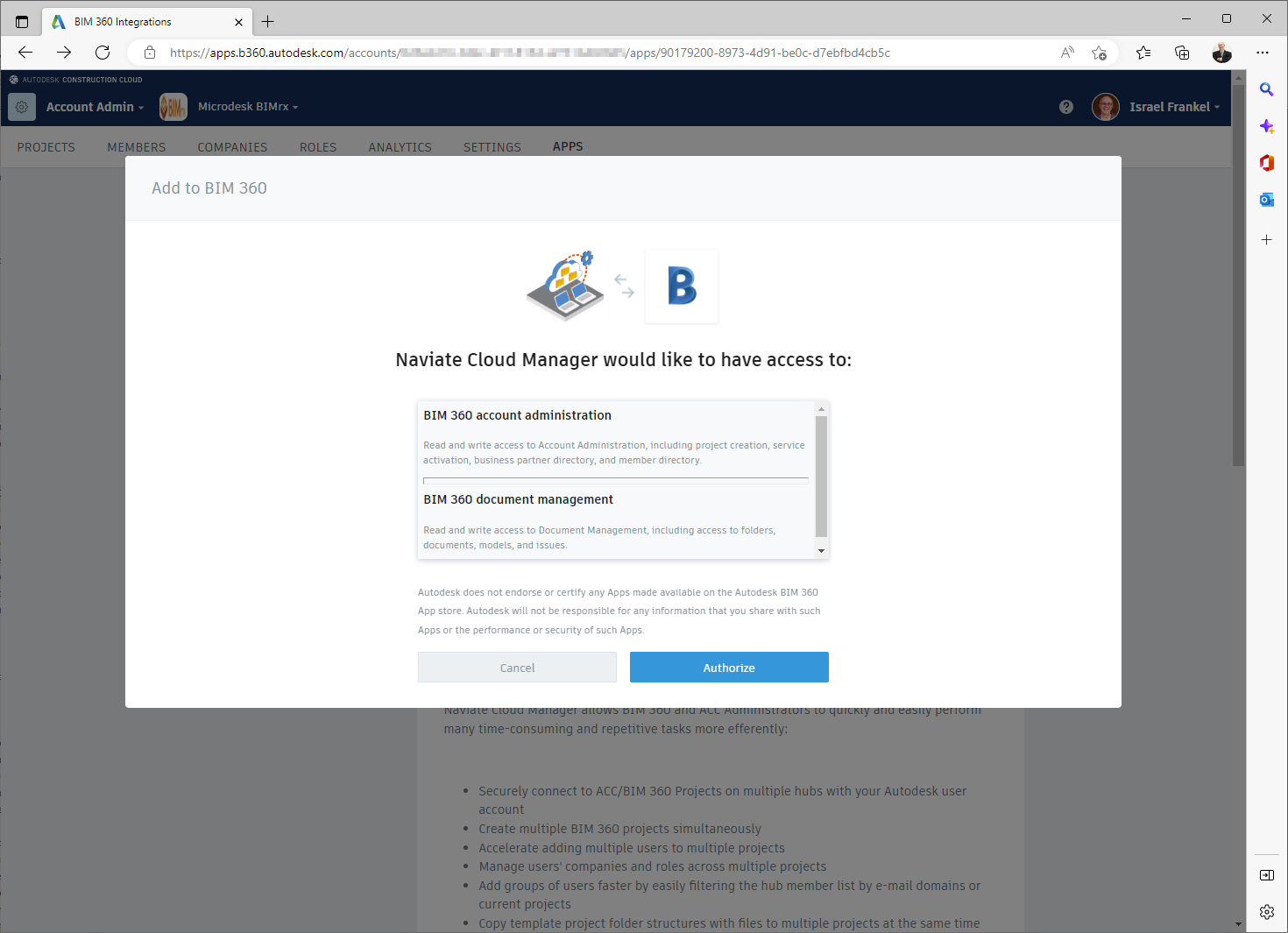This screenshot from the BIM 360 website captures a dynamic moment where a user interacts with a pop-up dialog. In the forefront, the pop-up titled "Add to BIM 360" is prominently displayed, containing an icon of two laptops with a cloud above them and a letter 'B' beside it. The text below reads, "Navigate Cloud Manager would like to have access to," followed by options for "BIM 360 Account Administration" and "BIM 360 Document Management." Users are given the choice to "Cancel" or "Authorize."

In the background, partially obscured by the pop-up, the site’s layout is visible. It shows an account amendment section, accompanied by relevant user information. Below this section, several navigable tabs are listed, including "Projects," "Members," "Companies," "Roles," "Analytics," "Settings," and "Apps." There is a large text box present, but its content is grayed out and not easily discernible. The overall interface offers a glimpse into the structured and user-centric design of BIM 360.